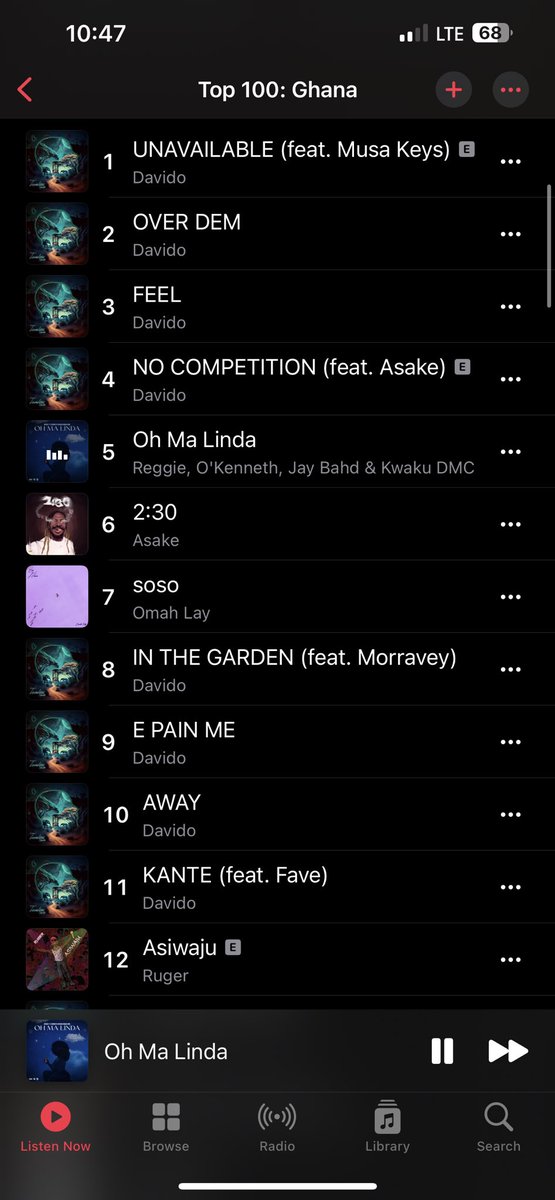The image depicts a smartphone screen displaying a music app against a black background. At the top of the screen, the time reads 10:47 on the left, while the right corner shows the icons for battery at 68%, signal strength, and LTE connectivity. The main focus of the screen is the "Top 100 Ghana" music chart, prominently displayed at the top. The title "Top 100 Ghana" is aligned to the height of the screen.

On the right side of this title, there is a red plus icon followed by a red three-dot menu icon. On the left side of the title, there is a red back button. The chart lists the top 12 songs, detailed as follows:

1. "Unavailable" by Davido
2. "Overtime" by Davido
3. "Failed" by Davido
4. "No Competition" by Davido
5. "Omalinda" by Reggie, Okenet, Jay, Bart, and Kwaku the MC (currently playing)
6. "Too Dirty" by Asake
7. "Soso" by Omalei
8. "In The Garden" by Davido
9. "E-Pain Me" by Davido
10. "Away" by Davido
11. "Cancer" by Davido
12. "Asiwachu" by Ruga

At the bottom of the screen, the music app's navigation bar features icons labeled "Listen Now," "Browse," "Radio," "Library," and "Search." The "Listen Now" icon is highlighted in red, indicating that it is currently active.